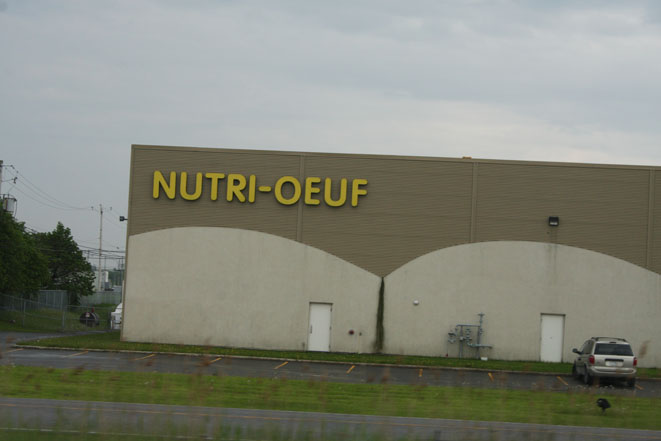In this dim, gray-lit daytime scene, we observe the rear side of a large business building characterized by its flat, squared-off architecture. The structure is primarily tan and brown, with prominently displayed yellow relief letters spelling out "N-U-T-R-I-O-E-U-F." Along the exterior, two white back doors are visible, accompanied by gas plumbing fixtures. Below the building, a parking lot stretches out, hosting a single gray car parked nose inward. The foreground reveals a road, and the sky overhead is covered in a blanket of gray, overcast clouds, adding to the overall muted atmosphere of the scene.